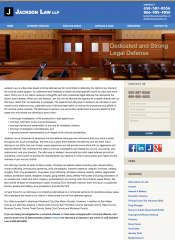The image depicts a website for Jackson Law, LLP. The overall design is somewhat blurry, making specific text difficult to read, but certain elements are discernible. At the top of the webpage is a blue banner. On the left side of this banner, there's a black square with a white "J" inside it, adjacent to the text "Jackson Law, LLP." To the right side of the banner, there is small print, accompanied by two phone numbers.

Below the banner, there are six tabs aligned horizontally, which likely serve as navigation links for the website. At the center of the page, there's a large media image displaying the words "Dedicated and Strong Legal Defense," overlaid on a depiction of two courtroom doors with wooden paneling visible on the walls and a faint glare on the floor.

Further down, the website contains several paragraphs of text, presumably providing more details about the firm's services, ethos, or case studies. On the right side of the webpage, there are additional phone numbers within a boxed section. This area also includes some information, social media icons, and a list of bulleted links for easy navigation.